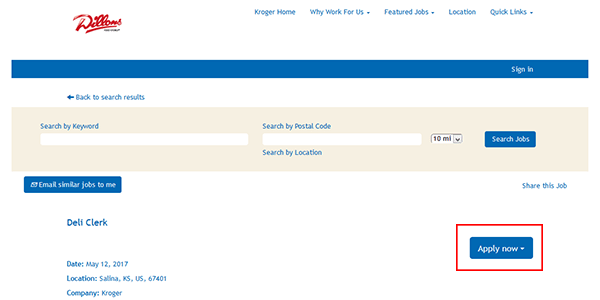This is a cropped screenshot of the job search portal for the grocery store chain, Dylan's. The image has a white background and prominently features the Dylan's logo in the top left corner. On the top right of the header, there are navigation links in a blue font, including "Kroger Home," "Why Work For Us," "Featured Jobs," "Location," and "Quick Links." Directly below this header is a blue bar with a "Sign In" option on the far right in small white letters.

Underneath the header, on the left side, there's a blue link labeled "Back to Search Results" accompanied by a small arrow pointing to the left. Below this link is a large, light pink box serving as the search area.

At the top of this search area, the text "Search by Keyword" is displayed above a long text box. To the right of this, there is another prompt labeled "Search by Postal Code" above a similarly large text box. Beneath the keyword search box, the words "Search by Location" can be found next to a small drop-down menu set to "10 miles," allowing users to filter job search results by distance.

Adjacent to the location drop-down menu is a large blue "Search Jobs" button. Beneath this light pink search area, on the bottom right, there's a text link that reads "Email Similar Jobs to Me," followed by a listing for a "Deli Clerk" position. On the far right, there is an "Apply Now" option highlighted by a large blue button, which is further emphasized by a red box edited around it to draw attention.